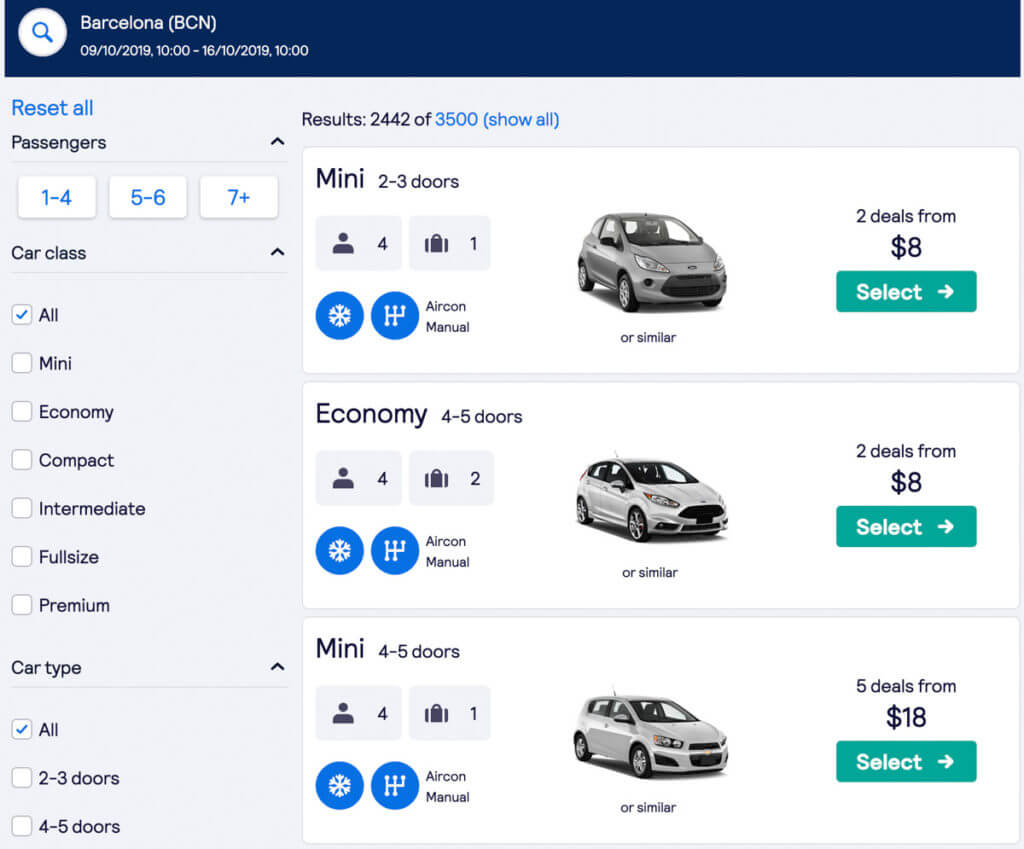The image appears to be an advertisement for a car rental service or possibly a ride-sharing service like Uber. At the top of the image, a blue border spans the width of the image, containing a white circle with a search icon in it. To the right of the search icon and still within the blue border on the left, the text "Barcelona (BCN)" is displayed. Below this, in a smaller font, the dates "09/10/2019" and "10:00 - 16/10/2019, 10:00" are provided, indicating the rental period from September 10, 2019, at 10:00 to September 16, 2019, at 10:00.

Moving into the main section of the image, a menu runs down the left-hand side. At the top left of this menu, "Reset All" is written, followed by "Passengers" options categorized into "1 to 4", "5 to 6", and "7 plus". Further down, the "Car Class" section allows the user to choose between different car classes with options such as "All", "Mini", "Economy", "Compact", "Intermediate", "Full Size", and "Premium". The "Car Type" section follows, showing that "All" is currently selected but also offering options for "2 to 3 doors" and "4 to 5 doors".

The main part of the image showcases the search results displaying different car options, including "Mini", "Economy", and another "Mini". This area on the right likely shows the cars matching the selected criteria from the menu on the left.